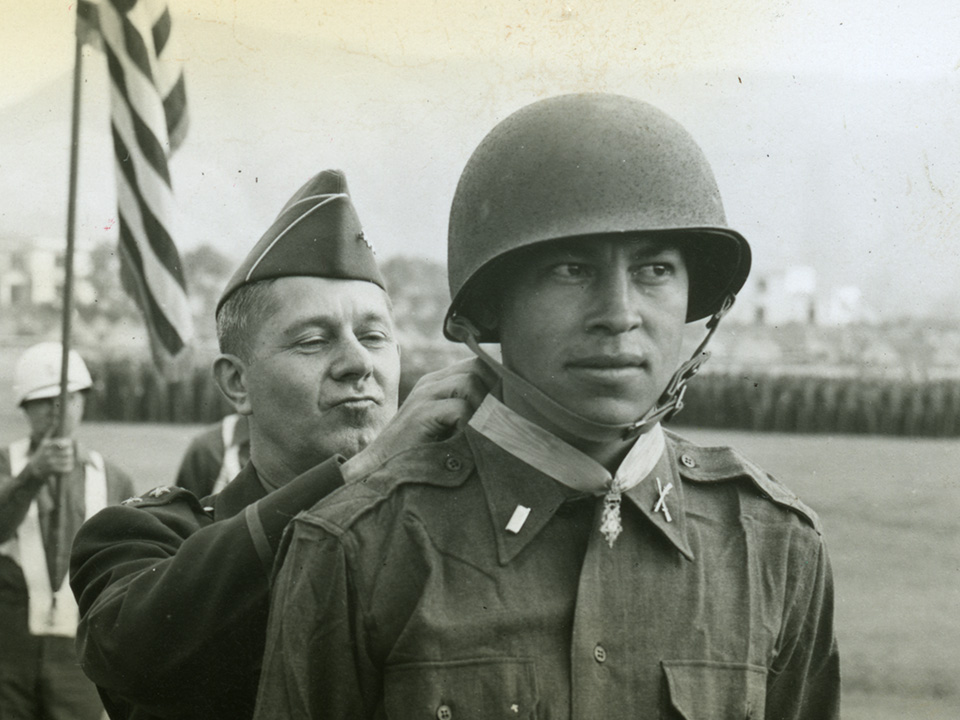This detailed black-and-white photograph captured outdoors showcases a poignant military scene. In a close-up view, an African American soldier, possibly of high rank like a captain, stands solemnly as he receives a medal from a white, middle-aged, two-star general. The general, positioned behind the soldier and slightly to his right, is intently affixing the medal around the soldier's collar. The captain gazes to his left, imbuing the moment with a sense of introspection.

The general appears pleased, his triangular-shaped hat suggestive of ceremonial attire rather than battlefield gear. The honor guard, poised just left of the soldiers, holds a prominently visible American flag, the bottom portion hanging down from the pole he supports. Although the honor guard's helmet is oval-shaped, resembling those used for protection, it contrasts with the general's headgear, underscoring the different roles and statuses within this assembly. 

In the unfocused background, a formation of soldiers stands at attention, mere silhouettes observing the prestigious moment from afar. The entire tableau solemnly captures a significant military commendation, reflecting both the gravity and honor of the occasion.